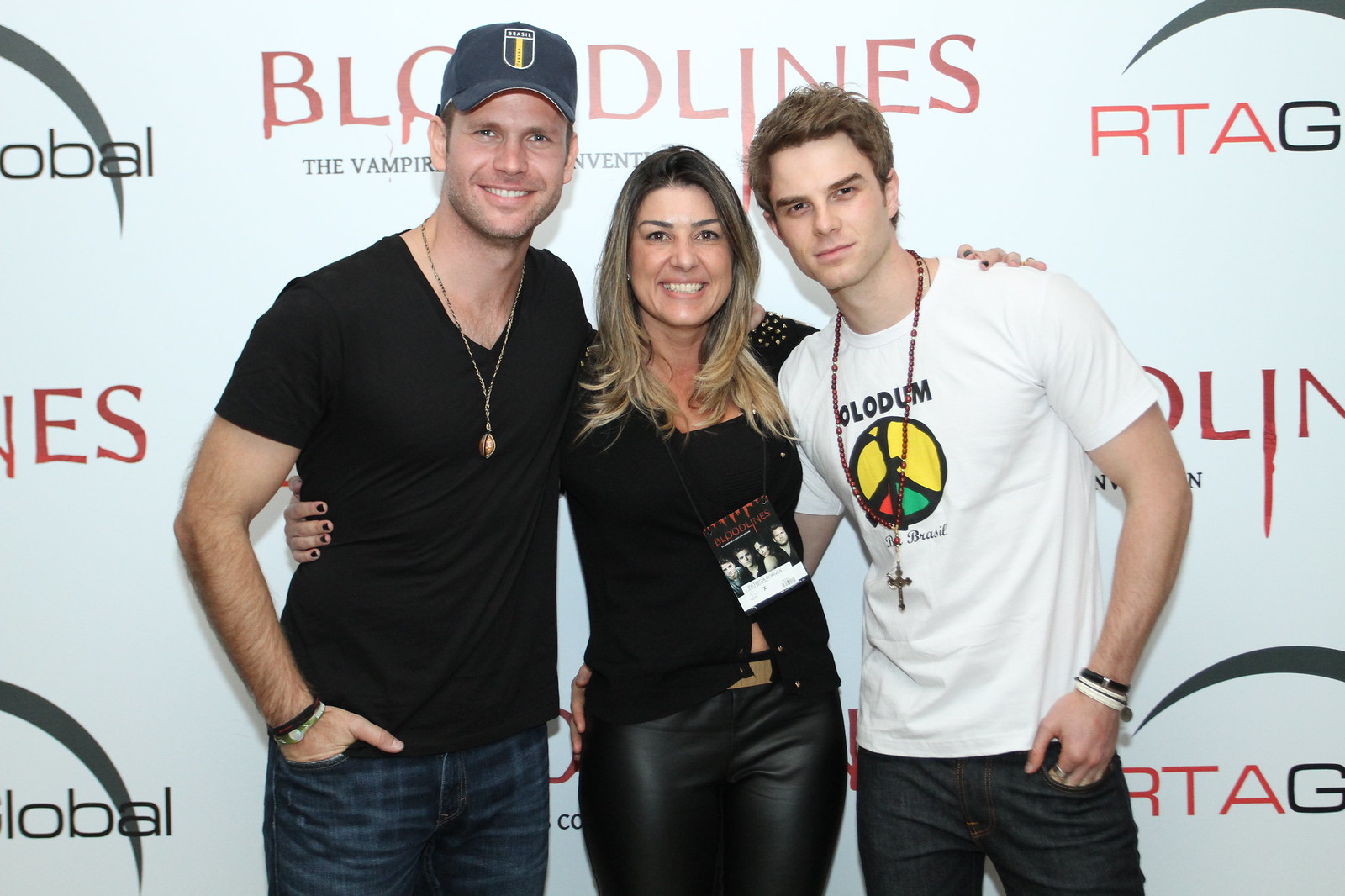In this vibrant image, set against a white background emblazoned with the repeated logos "RTA" and "Bloodlines," featuring blood dripping from some letters, three people pose together, suggesting a red carpet or event setting. Starting from the left, a taller man wearing a blue baseball cap, black v-neck t-shirt, and dark blue jeans stands with his right hand in his pocket, his left arm wrapped around the woman beside him. This woman, in the center, dons a black dress, with her long blonde hair cascading below her shoulders. She embraces both men warmly, smiling brightly. On her other side, a slightly shorter man sports a white t-shirt featuring a peace symbol with yellow, green, and red sections, along with a cross necklace. He pairs this with black jeans. All three appear Caucasian, radiating camaraderie and joy against the detailed and intriguing backdrop.